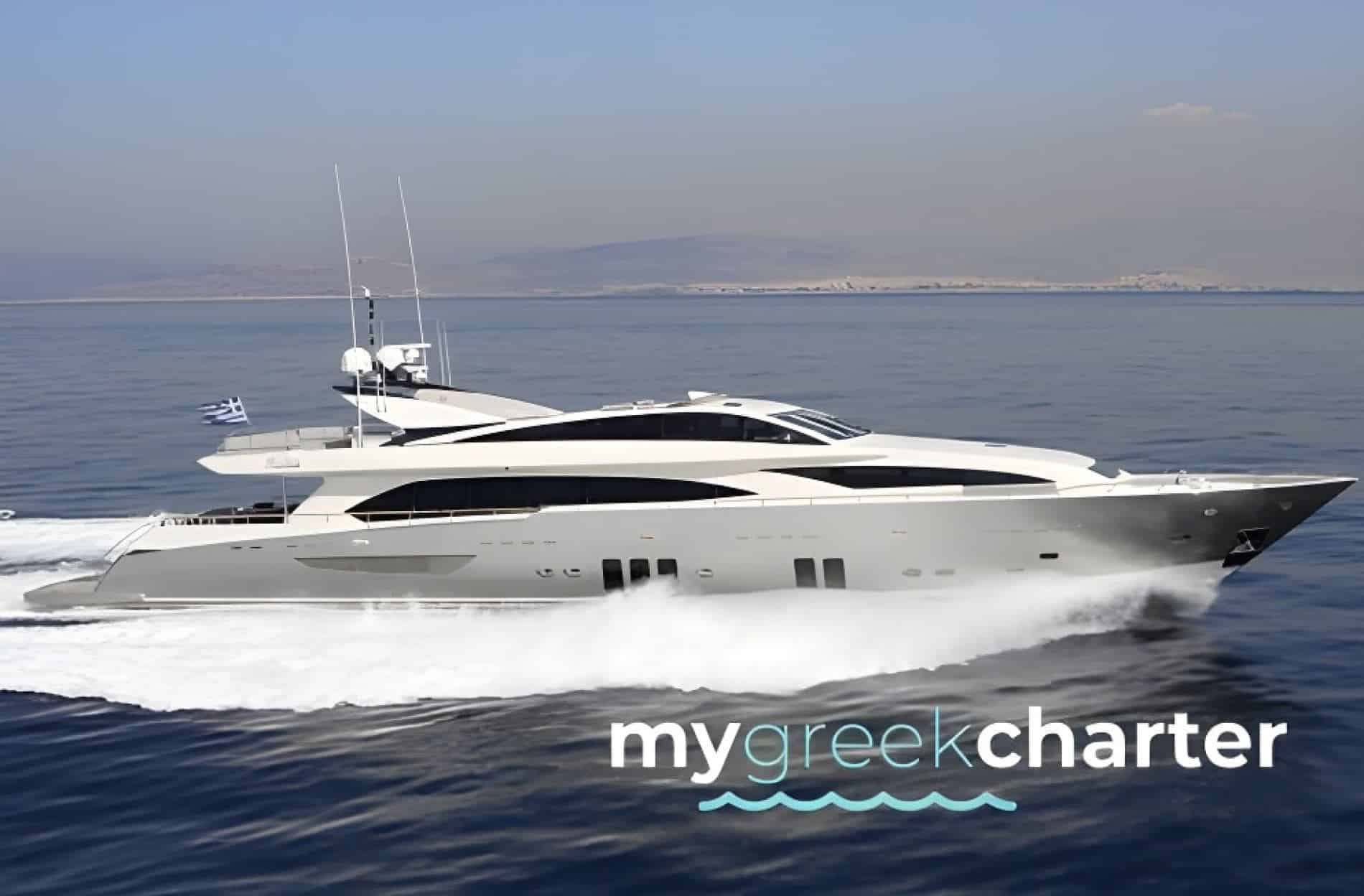A pristine white yacht with sleek black-tinted windows glides through azure waters, leaving frothy white wake in its path. The Greek flag flutters at its stern, suggesting a voyage through the Aegean Sea. In the background, a rugged island with rocky hills rises majestically from the water, completing the picturesque Mediterranean scene. In the bottom right corner of the image, an elegant caption reads "my Greek charter" in English, with the word "Greek" highlighted in light blue. This text overlays a subtle background of water and the yacht's reflection, while underneath "Greek," a delicate line drawing of water ripples adds a charming touch. The yacht is clearly identified as a rental, inviting onlookers to dream of their own Greek adventure.